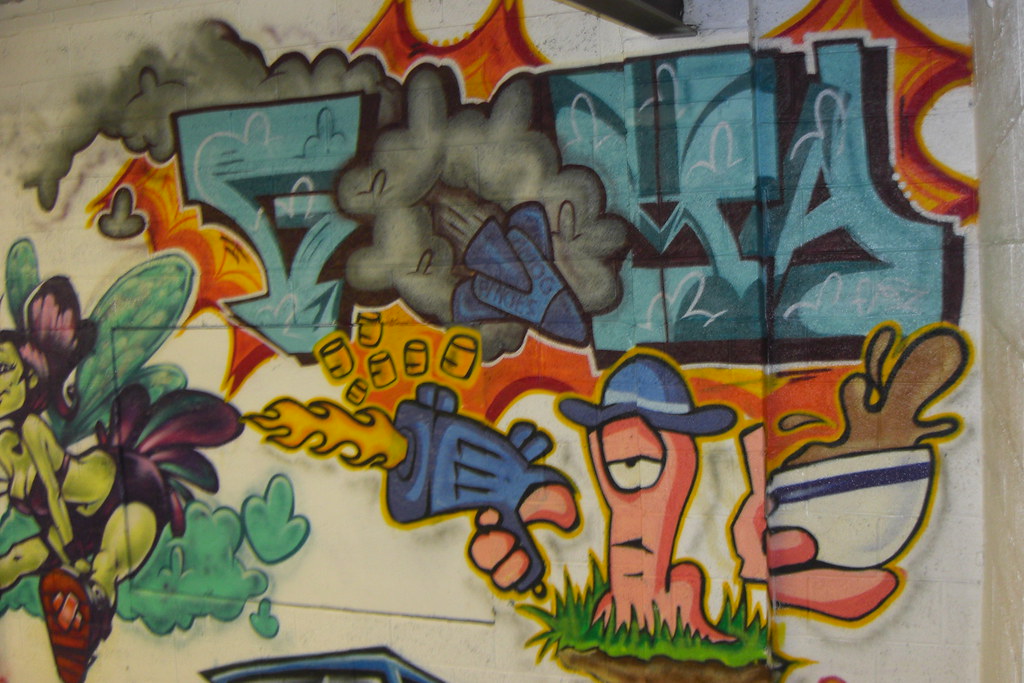The mural in the image is a vibrant and eclectic piece of graffiti painted on a white brick wall, potentially created by multiple artists due to its diverse styles. Dominating the scene is a cartoonish, worm-like character adorned with a blue hat. This character intriguingly has an eyeball painted on its nail and appears to be using hands that are not attached to its body. With its right hand, it wields a blue firearm that's actively firing, releasing bullets and flames from the barrel. In its left hand, it holds a white ceramic cup with a blue ring, spilling some of its presumably tea contents. To the left of this character is a green-skinned fairy with turquoise wings, brown shoes, and a purple outfit, presenting a whimsical contrast.

Above the characters, bold blue graffiti phrases are emblazoned, featuring a distinctive 'O' character that resembles a smoke cloud pierced by a small rocket. This graffiti is framed by a striking spiky border in orange and red hues. Additionally, at the bottom of the mural, there is a peach-colored alien creature with a blue hat, seemingly sitting on grass while holding a bowl of brown liquid, perhaps soup, and also spraying a blue gun with fire at the end. A sense of chaotic yet playful energy pervades the scene, making it a rich tapestry of colors and characters with intricate, imaginative details.